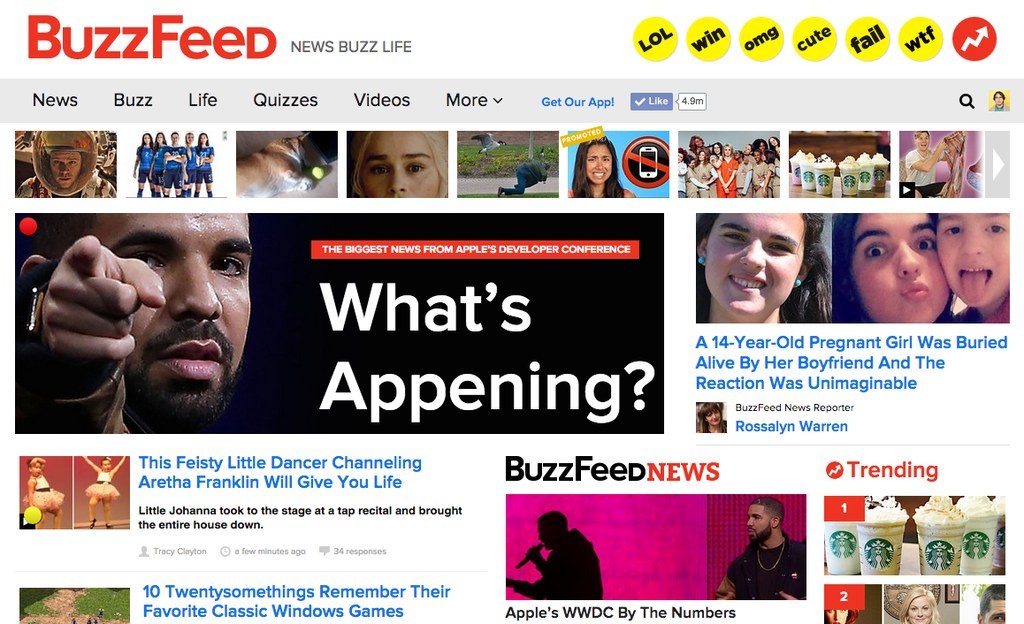On the BuzzFeed website, the BuzzFeed logo is prominently displayed in red, positioned in the top-left corner. The page is filled with various thumbnails and images corresponding to different news stories. The main headline features a black background with an image of a man pointing his index finger, accompanied by the text "What's Happening: The Biggest News from Apple's Developer Conference."

Adjacent to this, there is a thumbnail showing a young girl, with a caption beneath it that reads, "14-Year-Old Pregnant Girl Buried Alive by Boyfriend - The Reaction Was Unimaginable." Other prominent news stories include one about "This Feisty Little Dancer Channeling Aretha Franklin Will Give You Life," and an article titled "10 20-Somethings Remember Their Favorite Classic Windows Games."

Trending stories are highlighted, with the number one story related to Starbucks, featuring an image of four Starbucks cups topped with whipped cream. At the top of the page, several yellow circles containing black text label various reactions, including "LOL," "WIN," "OMG," "CUTE," "FAIL," and "WTF."